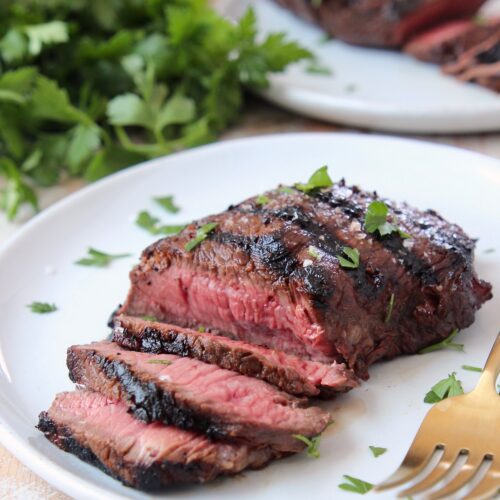The image features a medium-sized, medium-rare steak, beautifully arranged on a white, subtly curved plate. The steak, with its seared exterior and pink interior, presents clear grill marks indicating it was cooked on a grill. The main fillet remains intact, but three neatly cut slices are stacked towards the front of the plate. Scattered around the steak are small, decorative pieces of parsley or cilantro, adding a touch of green. A gold fork, only partially visible, lies next to the steak. In the upper left corner of the image, there’s a generous bunch of fresh cilantro or parsley directly on the table. The background reveals a slightly blurred second white plate with a similarly arranged and cooked steak, enhancing the primary focus on the steak in the foreground. This detailed arrangement highlights the meticulous preparation and presentation of the dish.